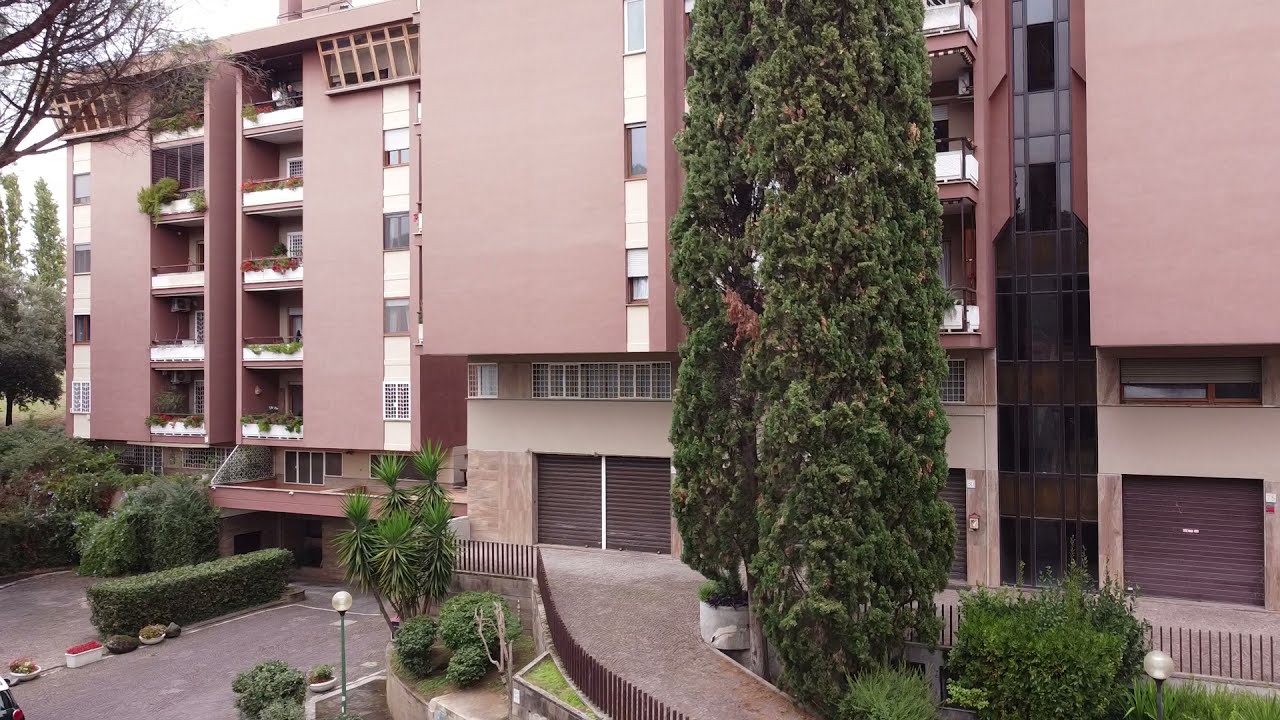This horizontally oriented photograph captures a large brown apartment complex—possibly a condominium or hotel—spanning six to seven floors. The building features multiple balconies, each adorned with lights and hanging plants, offering residents outdoor spaces. The structure includes several brown garage doors and glass-framed sections running vertically along one side. In front of the building, meticulously manicured hedges are shaped into a long rectangle, accompanied by palm trees and other well-maintained trees, including two prominent tall ones near the center-right that partially obscure some balconies. The scene, taken during the daytime with a cloudy sky visible in the upper left corner, also shows a small road lined with a brown fence, paved walkways, and white posts. In the distance, more trees can be seen, adding to the picturesque setting.